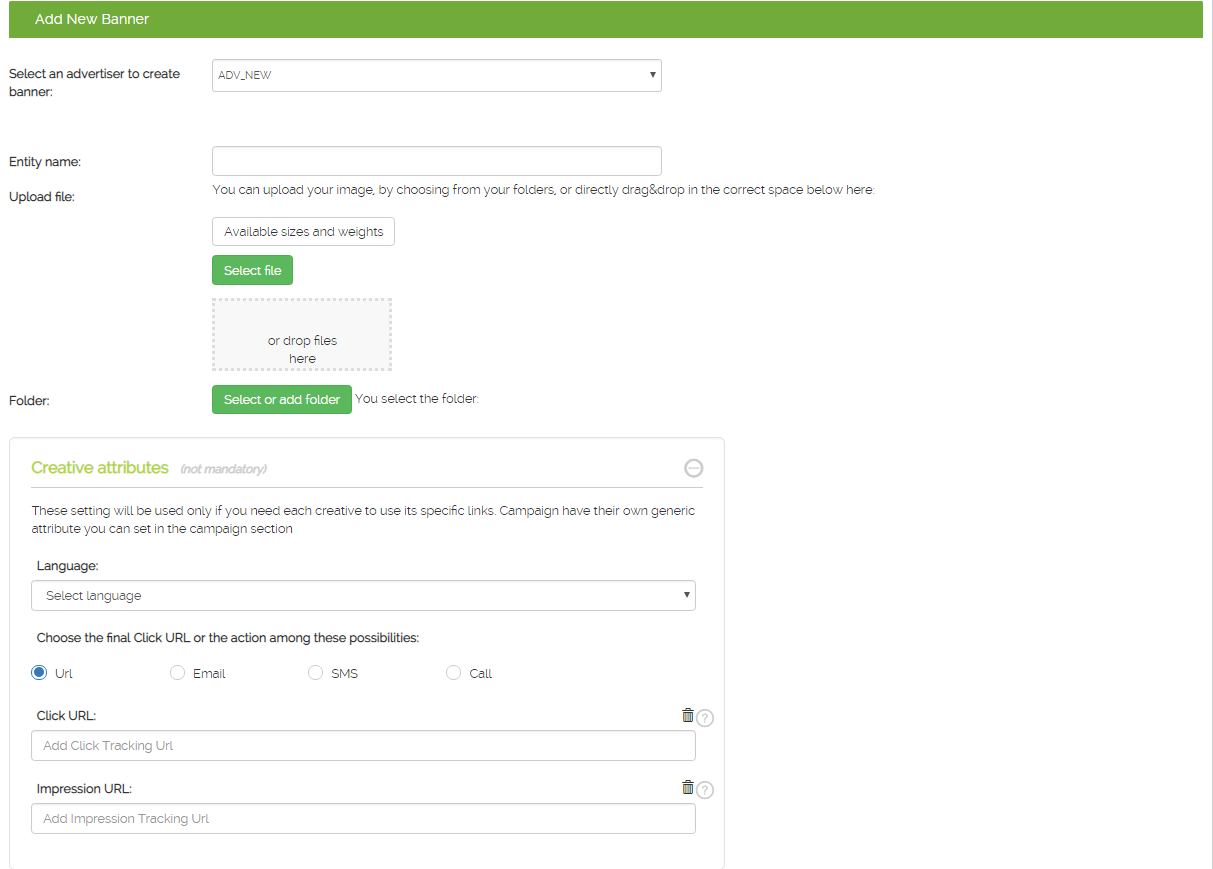In this image, we see a detailed online form designed for adding a new banner within an advertising platform. At the top of the page, there is a section prompting the user to "Add New Banner." Below this header, a series of input fields and dropdown menus guide the user through the banner creation process.

The first field is labeled "Entity Name," where users can input the name of the entity to which the files will be uploaded. Following this, there's an "Upload Files" option that allows users to choose files to include in the banner.

Next, the user is prompted to select a folder or add a new one in the "Folder" field. There is a section for "Creative Attributes," which is optional and meant for setting individual creative links if necessary. The form clearly states that these settings will only be used if unique links for each creative are required.

Further down, there is a "Campaign" section noting that generic attributes for campaigns can be set in the campaign section separately. 

For language preferences, there is a "Language" dropdown field to select the desired language for the banner.

At the bottom, the form provides multiple options for the final click URL or action, offering choices such as URL, email, SMS, and call. By default, the "URL" option is checked. Within this section, users can add a "Click URL" for click tracking and an "Impression URL" for impression tracking.